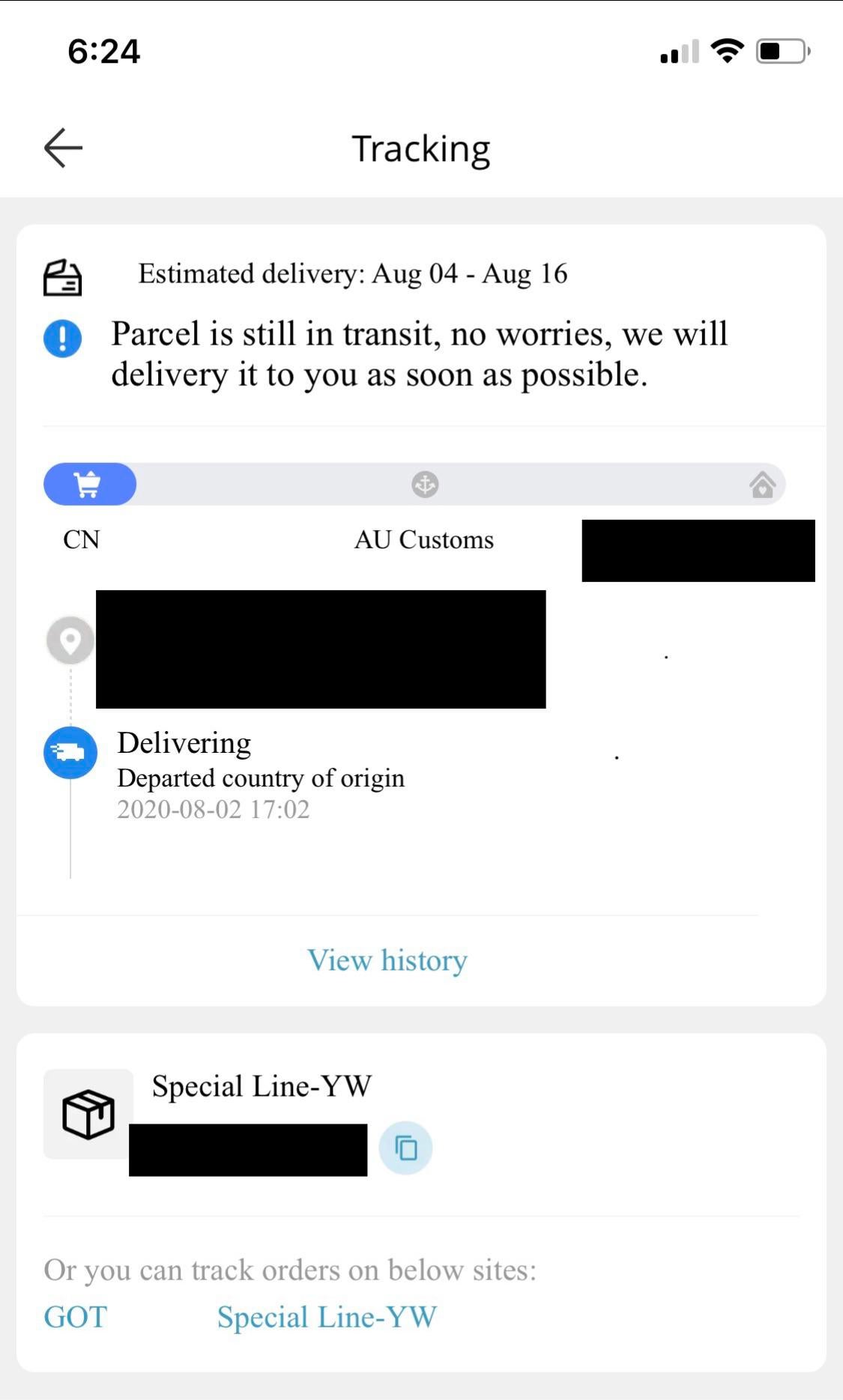The image appears to be a detailed screenshot from an Android device, showcasing a package tracking interface. At the very top, there is a thin black status bar. On the left side of this bar, black text indicates "6:24" on a white background, next to icons representing signal strength (two out of four bars), Wi-Fi connectivity, and a half-filled battery. Below the time "6:24," there is a black left-pointing arrow.

Midway through the image, the word "Tracking" is displayed in black text within a gray-rimmed box which has a white interior. Towards the upper left of this section, there is a black envelope icon next to the text "Estimated Delivery: AUG 04 - AUG 16" in black letters. Below this, a blue circle with a white exclamation mark contains the notification, "Parcel is still in transit. No worries, we will deliver it to you as soon as possible," written in black text.

Beneath this information, a long, gray navigation bar features a blue section with a white shopping cart icon. Other small logos are present, including a gray circled icon of a person opening a package in the center and a house icon on the far right. Below the blue section, the letters "CN" are centered under the person icon, while "AU CUSTOMS" appears below this, and a black redacted box occupies the far right.

Further down, a black location icon is separated by a thin gray line, adjacent to a blue circle with a truck icon to the right of which "Delivering" is written in black text. The next line reads, "Departed Country of Origin" in grey text, followed by "2020-08-02 17:02." At the bottom of this section, a phrase "View History" is written in blue text, separated by a faint gray line.

Towards the lower section, another white rectangular box with a gray square inside it contains a black box icon. To the upper right of this box, it says "Special Line - YW" with a long black rectangle redacting information below it. On the right, there is a faint blue circle with an icon of two blue-outlined papers, one atop the other. The text "Or you can track orders on the below sites" appears in gray towards the section's bottom left. In the lower-left corner, "GOT" is printed in blue, followed by "Special Line - YW" also in blue, with "YW" in all caps.